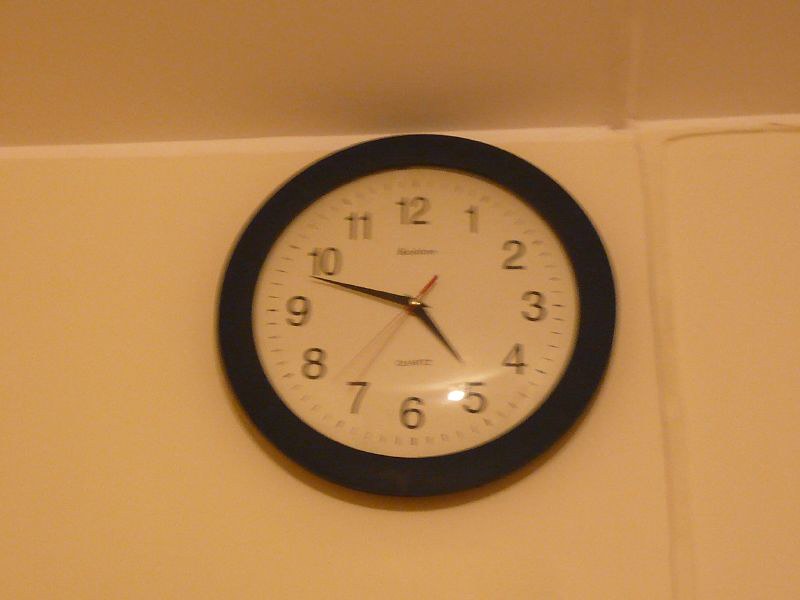In this image, we're inside a room that appears to have a beige-orange hue, likely due to a filter giving the entire scene an orange cast, as if under a specific lighting condition. The focal point is a clock on the wall, framed in black, though it's unclear whether the frame is made of wood or plastic. The clock, showing 4:48 and 37 seconds, has black hour and minute hands and a red second hand. The numbers on the clock face range from 1 to 12. The room's structure suggests it is built from stone or cement blocks, with visible lines on the walls that may indicate the presence of pipes above or within the wall.